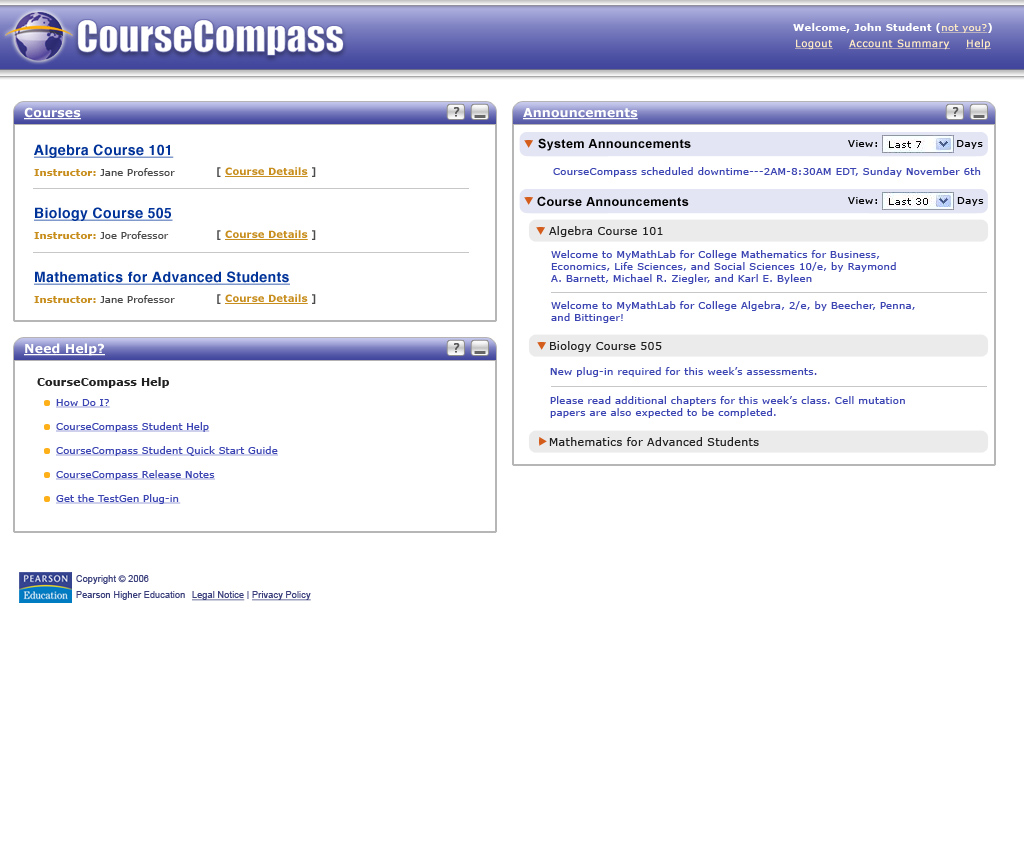*Caption: A detailed screenshot of an educational platform's dashboard filled with important information.*

The top of the bar features an Earth icon followed by an orange line, with options including "Course Compass," "Welcome John (Student)," and "Not You? Logged out." The "Account Summary" and "Help" sections are also visible.

There are multiple courses listed:
1. **Algebra Course 101**
   - **Instructor:** Jane Professor
   - **Details:** Course details accessible.

2. **Biology Course 505**
   - **Instructor:** Joe Professor
   - **Details:** Course details accessible.

3. **Mathematics for Advanced Students**
   - **Instructor:** Jane Professor
   - **Details:** Course details within brackets.

A blue section labeled "Meet Help" and a question mark icon prompt further assistance. Another section titled "Course Compass Help" offers a "Student Quick Start Guide," "Release Notes," and an option to "Get the Test Gen Plugin."

At the bottom, various administrative links are displayed: "Pearson Education," "Copyright 2006 Pearson Higher Education," "Legal Notice," "Privacy Policy."

**Announcements:**
- **System Announcements for the Last 7 Days:**
  - Course Compass scheduled downtime: 2 AM to 3 AM, Sunday, November 6th.
- **Course Announcements for the Last 30 Days:**
  - **Algebra Course 101:** "Welcome to My Math Lab for College Algebra 2," utilizing textbooks for mathematics in business, economics, science, and social sciences by Raymond A. Barnett, McCartney, Zepan, Connelly, and Byland.
  - **Logic Course 505:** Announcement for a new plugin required for this week's assessments. Additional readings on cell mutation papers are expected for completion.
  - **Mathematics for Advanced Students:** Consistent updates and details available.